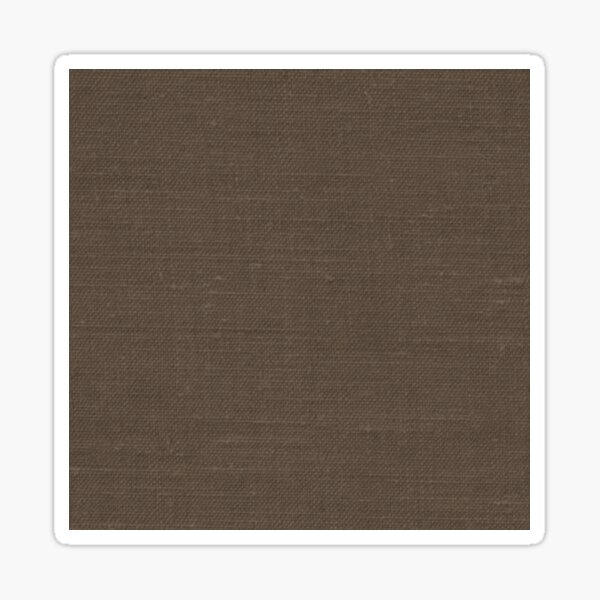The image depicts a sample of textured material, most likely fabric or carpet, featuring fine, brown horizontal and vertical textures that are subtle yet noticeable. The material, measuring approximately 4 inches by 4 inches, is carefully placed within a white border that frames the square sample. The texture, resembling a slightly rough fabric or a carpet with small dots or pilling, suggests a tactile quality of decent craftsmanship. The overall presentation, with the clean white border, highlights the brown texture at the center, emphasizing the material's intricate detailing and finish.